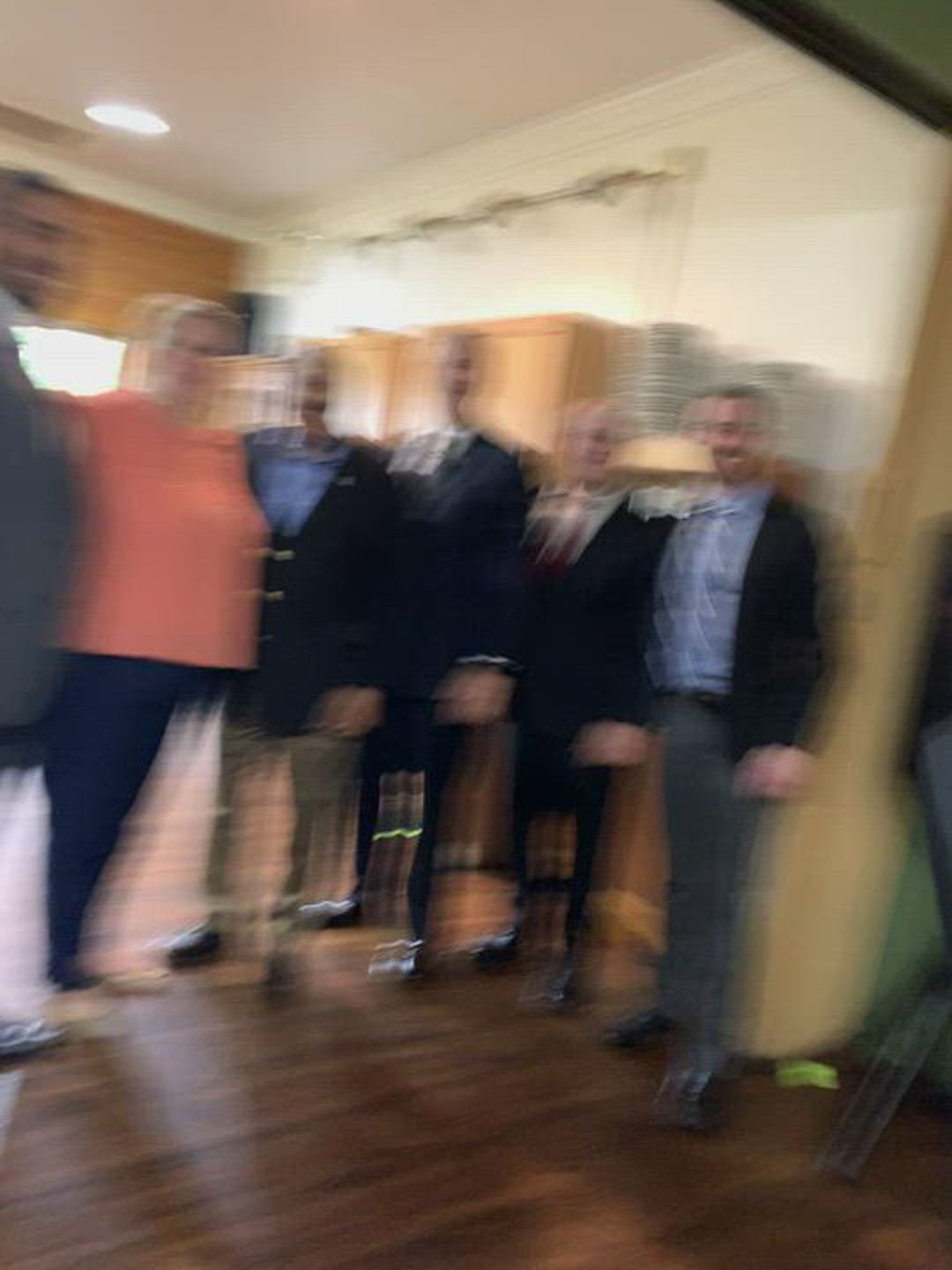A group of people, mostly men dressed in suits, are smiling at the photographer during what appears to be a work-related event or gathering. Among the group is a woman standing out in blue jeans and an orange, sleeveless top. She has her hair pulled back in a ponytail. The setting is bright and inviting, with ample sunlight streaming through a window behind them, suggesting it is daytime. The room's flooring is wooden and the walls are painted a neutral beige, adding to the warm atmosphere.